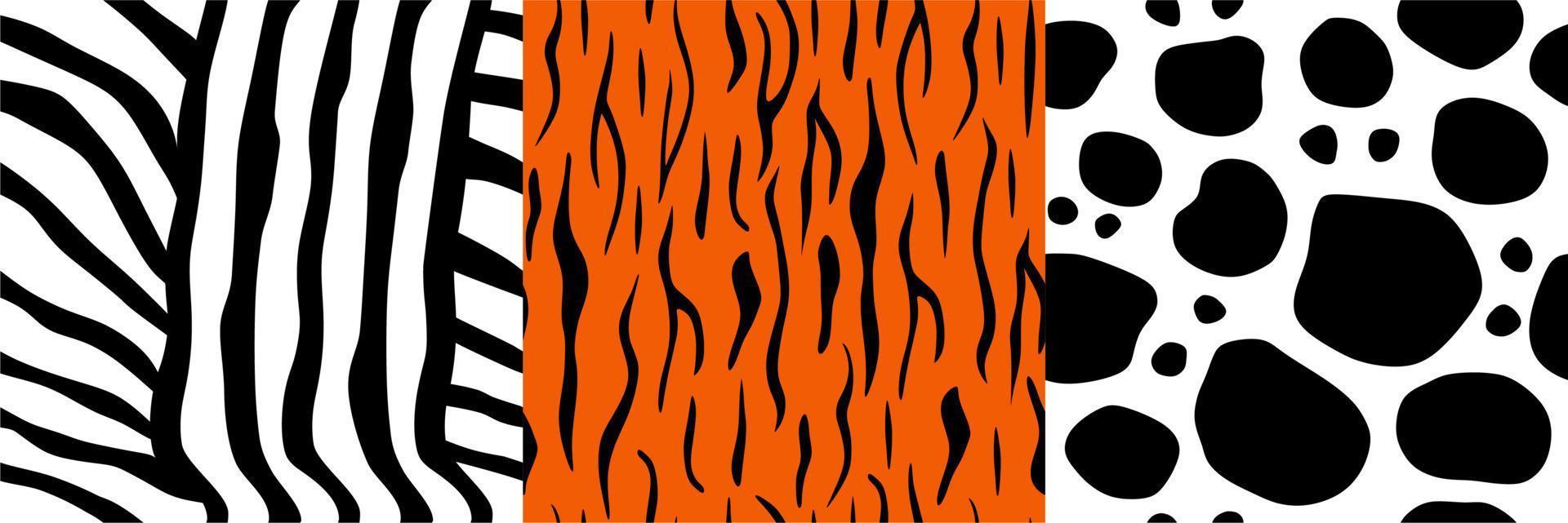The image displays three distinct panels, each evocative of different animal prints and modern art. The far-left panel features a white background with five curving black vertical lines resembling a zebra’s stripes, extending horizontally from the outermost lines. The central panel showcases an orange backdrop adorned with irregular black vertical striations reminiscent of a tiger’s pattern, where the stripes nearly touch without actually connecting. The far-right panel presents a white background dotted with black circles and smaller circles nestled between them, suggesting the intricate pattern seen on a leopard's coat. These three panels, side by side, create a compelling visual contrast, highlighting the unique textures and coloration of each depicted animal pattern.